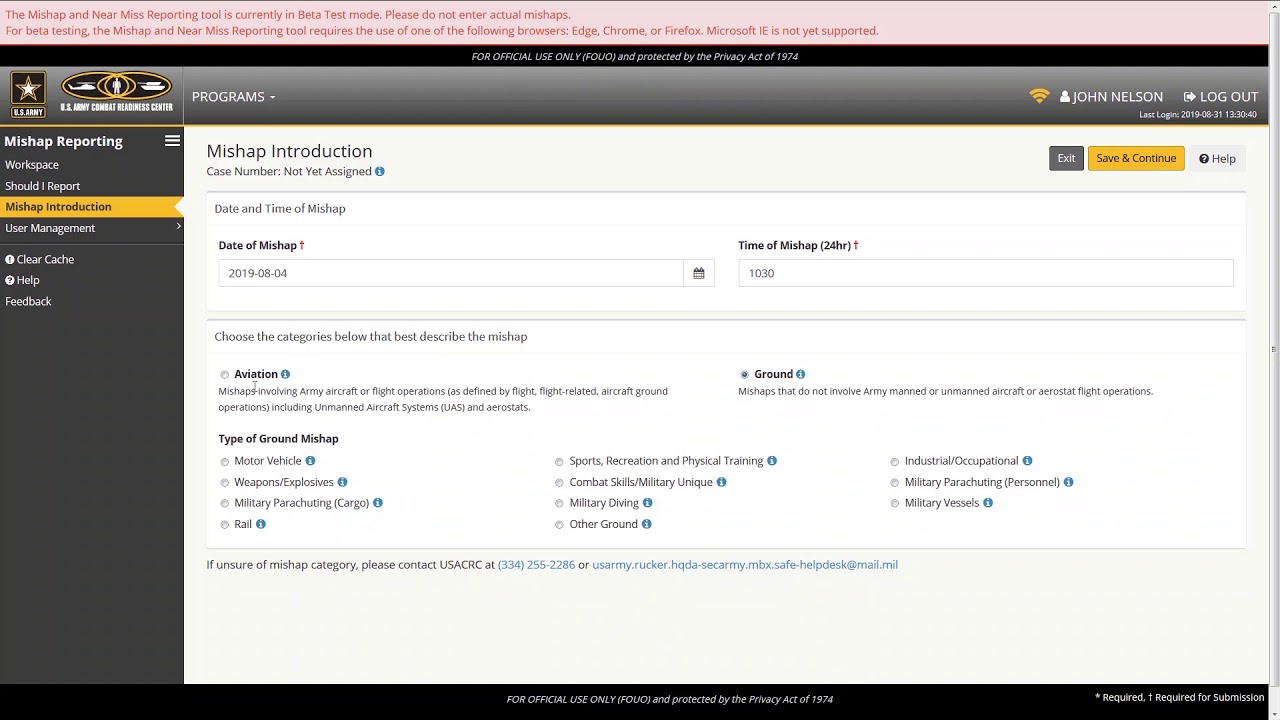Sure, here is a detailed and cleaned-up caption for the image:

---

This screenshot depicts the user interface of a beta version of the U.S. Army's mishap and near-miss reporting tool website. At the top of the page, a prominent pink banner features a message in darker pinkish-mauve print, stating: "The mishap and near-miss reporting tool is currently in beta test mode. Please do not enter actual mishaps." A second line on the banner informs users that for beta testing, the tool requires the use of one of the following browsers: Edge, Chrome, or Firefox, while noting that Microsoft IE is not yet supported.

Below the pink banner, a smaller black banner spans the width of the page, displaying an alert: "For official use only (F-O-U-O) and protected by the Privacy Act of 1974." 

Further down, a gray banner highlights the U.S. Army Combat Readiness Center with a drop-down menu labeled "Programs." To the right of this, a Wi-Fi signal icon indicates that the user, "John Nelson," is logged in, with their last login timestamped as 2019-08-31 at 13:30:40.

On the left side of the page, a sidebar starts with a gray background that darkens towards the bottom. It contains several menu items: "Mishap Reporting" (signified by three horizontal lines), "Workspace," "Should I Report," "Mishap Introduction" (highlighted in a yellow banner), "User Management," "Clear Cache," "Help," and "Feedback."

The central portion of the interface is a large white section surrounded by the gray banners. At the top, it reiterates "Mishap Introduction" and provides fields such as "Case Number: Not yet assigned," "Date and Time of Mishap," "Date of Mishap," and "Time of Mishap." Users are prompted to choose categories that describe the mishap, including options like "Aviation," "Ground," and sub-categories under "Type of Ground Mishap."

---

This caption offers a comprehensive and detailed description of the website's interface, effectively conveying the layout and specific details presented in the image.